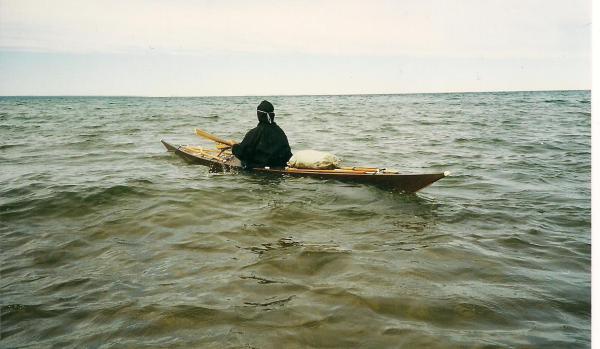In this image, a lone man is paddling a small canoe in what appears to be the open ocean. The water around him is murky, with a grayish-green hue, suggesting a somewhat muddy environment. The sky above is overcast, casting a gray pall over the scene, although no distinct clouds are visible. The man, whose back is turned to the camera, is fully clothed in black and has a band tied around his head. His oar is held in his hand as he navigates the calm, expansive waters stretching out endlessly to the horizon. Positioned in the canoe with him is a mysterious white bag. Additionally, a yellow rope is noticeable at the stern of the boat. There are no other people or boats in sight, emphasizing his solitude in this vast, serene expanse.